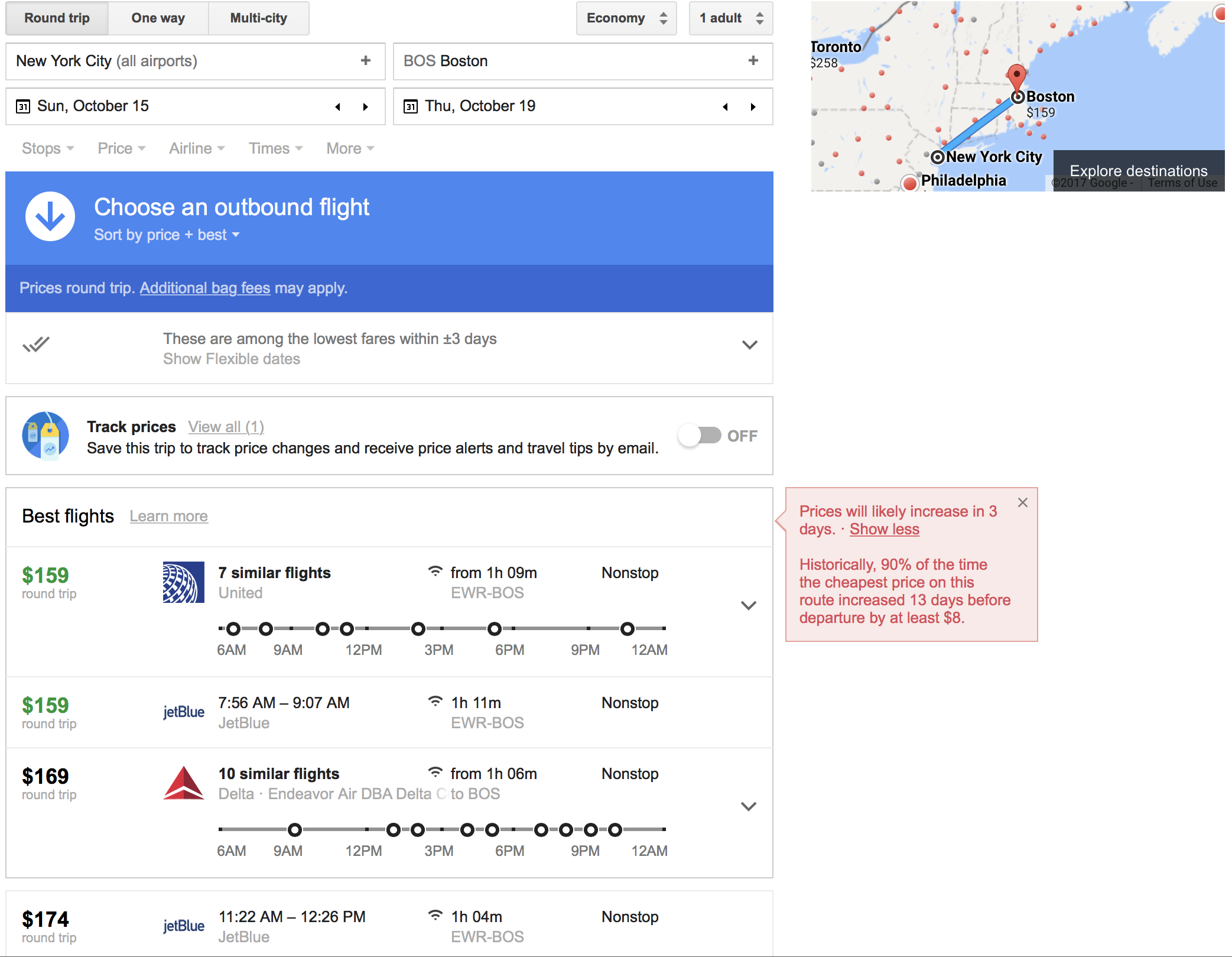The image displays a flight booking interface. At the top right, there is a round grey button labeled "One Way," followed by another button labeled "Multi-City." Next to these is a drop-down menu labeled "Economy" and another one labeled "1 Adult."

Below these options are four drop-down menus arranged in a grid format. The top-left menu is set to "New York City, All Airports," while the top-right menu is set to "BOS Boston." The bottom-left menu indicates the departure date as "Sunday, November 15th," and the bottom-right menu shows the return date as "Thursday, October 19th."

Beneath these menus, there are filter options for "Stops," "Price," "Airline," and "Times." Below these filters, there's a blue rectangular button labeled "Choose an Outbound Flight," accompanied by a white circle with an arrow pointing down, suggesting sorting options by price or best fit. Additionally, the text mentions that the prices are for round-trip tickets and that additional baggage fees may apply. It also notes that the displayed fares are among the lowest within a flexible date range of plus or minus three days.